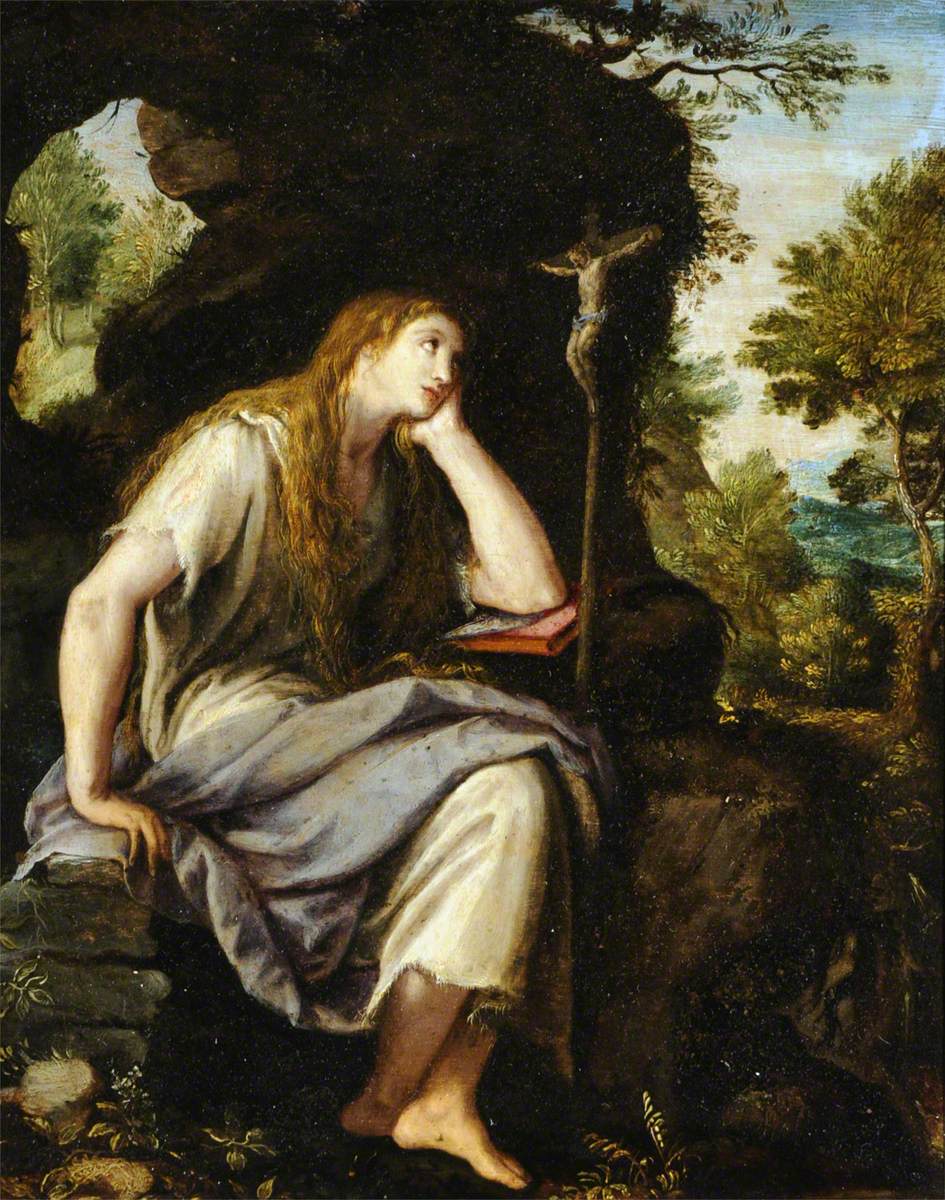The painting, reminiscent of works by the old masters and appearing notably aged, depicts a woman seated on a throne-like structure of rocks against a dark rock face. This detailed composition is rich with earthy browns and contrasts. The woman, barefoot and possibly weathered by time, displays a serene visage as she gazes contemplatively at a small crucifix bearing Jesus, positioned to her right. She wears a flowing white dress and a blue shawl draped over her thighs, and her long, reddish-brown hair cascades down to her waist. Her left hand rests thoughtfully under her cheek as her elbow supports a red book. The background features vivid blue skies and lush green trees visible through openings in the rock. A notable archway-like crevice is situated above her left shoulder, enhancing the scene's depth and natural setting. This masterfully detailed painting, with its interplay of light and shadow, evokes the timelessness of a four or five hundred-year-old masterpiece that one might expect to find in a museum.